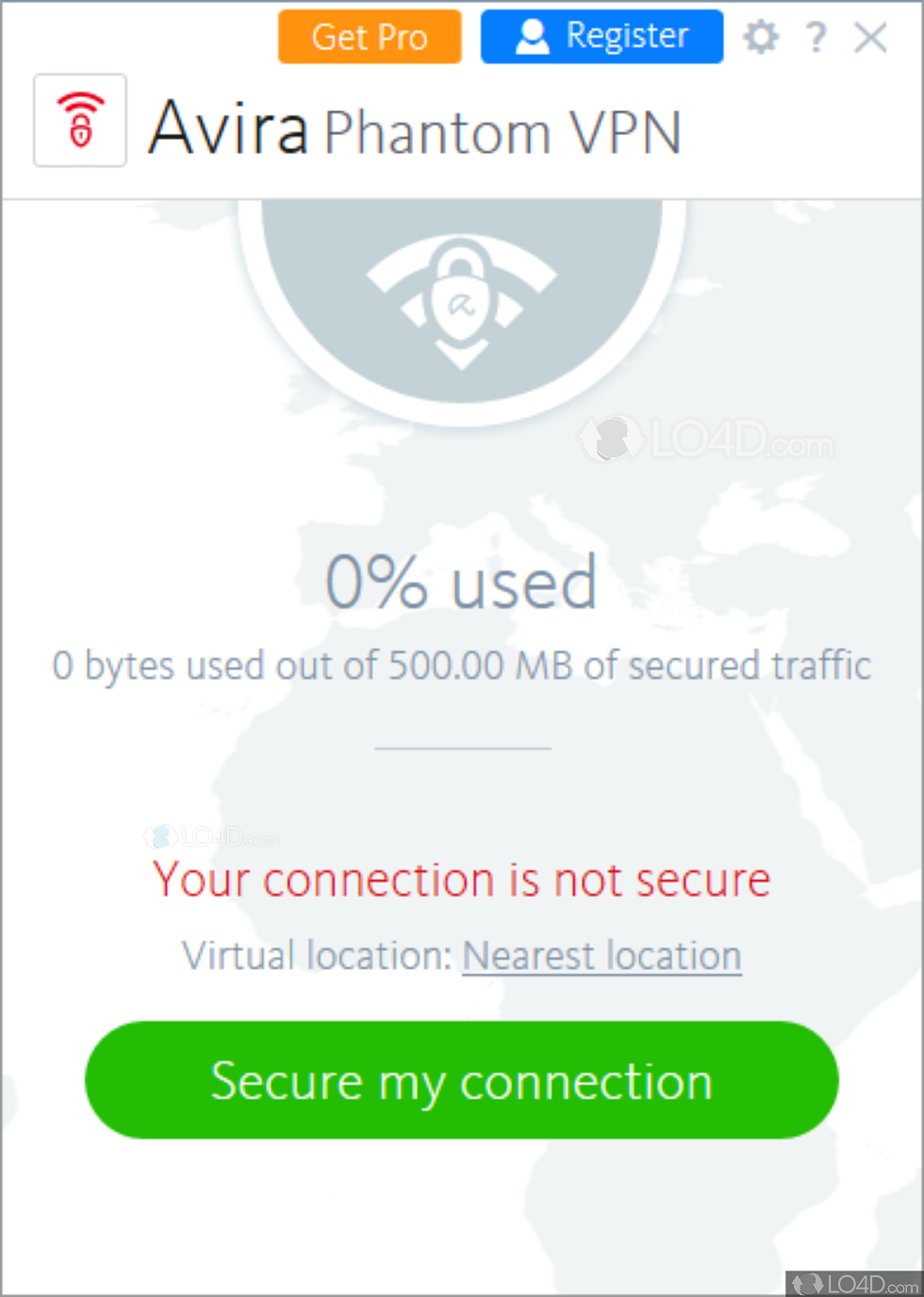Screenshot from a smartphone displaying the Avira app interface.

At the top, the header background is white. On the left, there is an orange rectangle with "GET PRO" written in white, and to the right of it, a blue rectangle with "REGISTER" written in white next to a white account icon. Below this header, "Avira" is written in black font, followed by "PHANTOM VPN" in gray.

On the left side, there is a red Wi-Fi icon connected to a padlock symbol, representing a secure private connection.

The main background is a mix of white and very light blue with some illustration. Below this, in light gray font, it reads "0% used." Beneath this, a red warning message says, "Your connection is not secure."

Finally, at the bottom, there is a green rectangle with rounded corners featuring the text "SECURE MY CONNECTION" in white.